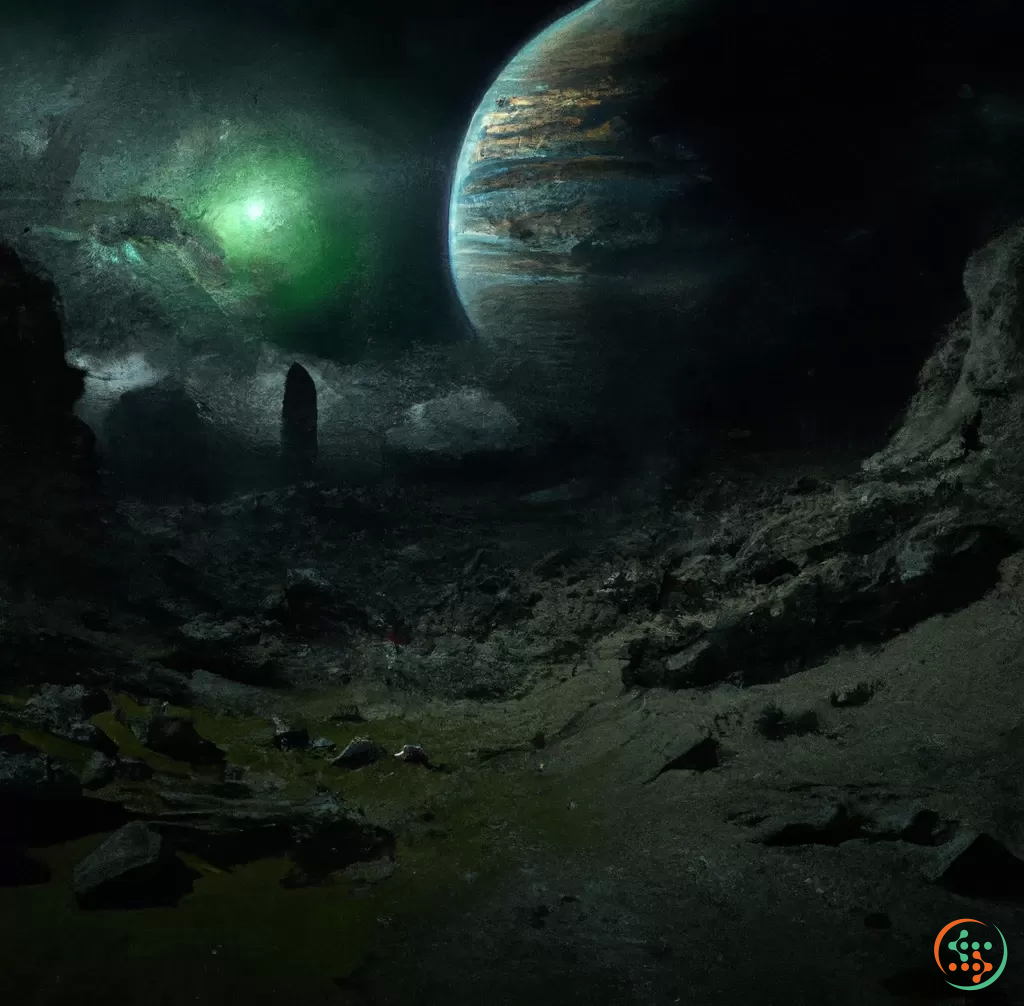The image is a vertically rectangular, multi-colored artistic print featuring a barren, rocky alien landscape primarily composed of dark gray and black hues, evoking a desolate and otherworldly feel. Dominating the upper right quadrant is a large planet that closely resembles Jupiter, positioned as if it is resting on the surface of another celestial body. Adjacent to it, in the distant sky, a faint green glow—possibly the sun—illuminates the scene, suggesting an outer space setting far within our solar system. The upper left corner features an enigmatic green glowing light, adding to the mystique. Scattered across the dark, rocky terrain are variously sized rocks. In the lower right-hand corner is a noteworthy symbol: a circle split into two half-circles, one red and one blue, containing two arrows—a blue one pointing left and a red one pointing right. The composition lacks any human presence, focusing solely on this stark extraterrestrial environment.